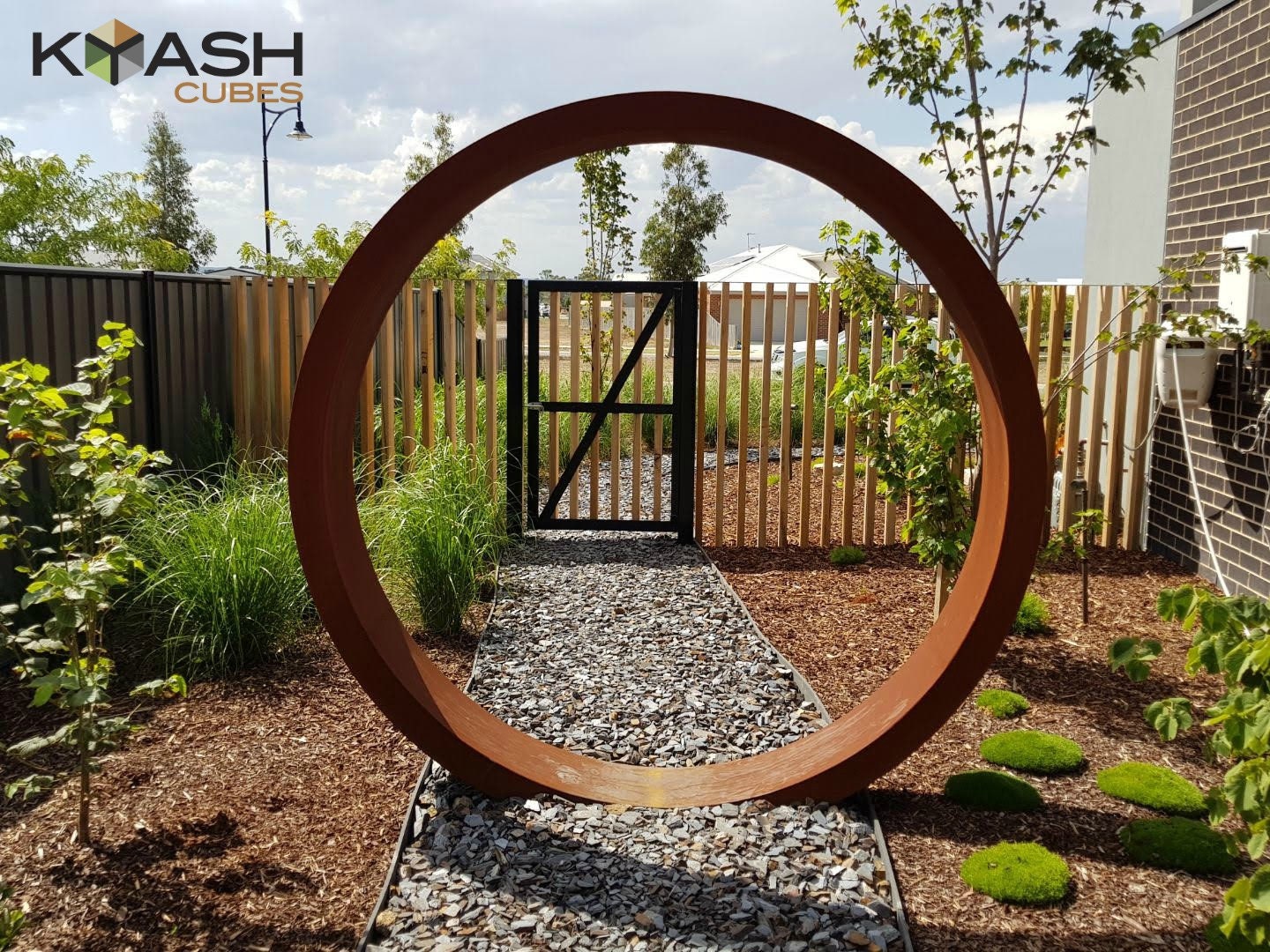This is an advertisement or informational outdoor image prominently featuring a landscaped area up against a brown brick building. At the top of the image, the text "Cash Cubes" is displayed, with an icon of a cube between "K" and "A-S-H." Dominating the middle of the scene is a large, hollow, circular metal structure, brown in color, set within a gravel walkway lined with metal strips. Surrounding this path are meticulously arranged flowerbeds covered in wood chips and mulch, featuring a variety of plants, including small shrubs, grasses, moss, and some young trees with green leaves. On each side of the walkway, there's a black fence leading to a gate made of wooden planks attached to two black posts. Beyond the fence, additional younger trees and the roof of a white structure are visible against a mostly cloudy sky.